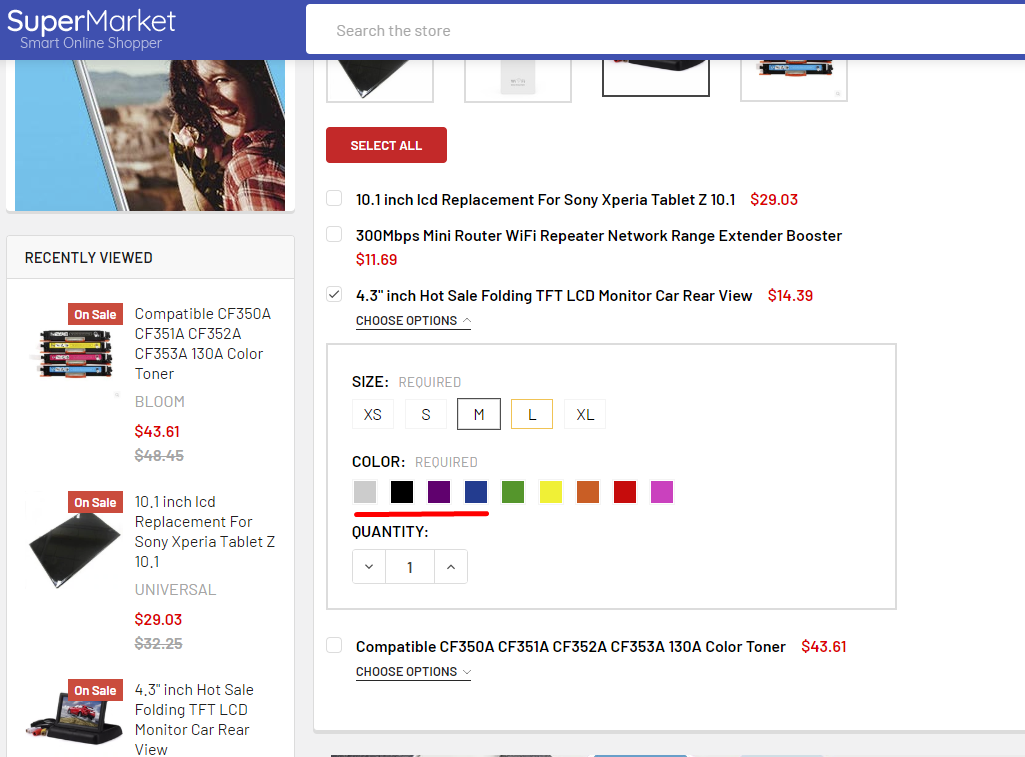A screenshot showcasing a supermarket's online shopping website. In the top left corner, the website's logo reads "Supermarket, Smart Online Shopper," alongside a search bar with the placeholder text "Search the store." Below the header, there is a promotional image featuring a woman in a plaid shirt.

On the left-hand column, a "Recently Viewed" section displays an assortment of items. The first item is an ink toner labeled "On Sale," with model numbers indicated for compatibility. The item description includes "Color Toner, Bloom" priced at $43.61 in red, with the original price of $48.45 crossed out below.

The next item listed under "On Sale" is a tablet screen replacement described as a "10.1 inch LCD Replacement for Sony Xperia Tablet Z 10.1, Universal," priced at $29.03 in red, down from $32.25.

Following this, another item on sale is a small monitor, specifically a "4.3 inch Hot Sale, Folding TFT LCD Monitor for Car Rear View." 

To the right, there is an option to "Select All" items, each accompanied by a checkbox. Of the items listed, only the box next to the rear view monitor is checked.

Below the item options, a section titled "Size Required" highlights "M" in black, with a follow-up section "Color Required" listing various color choices. Finally, a "Quantity" section indicates that the number one is selected.